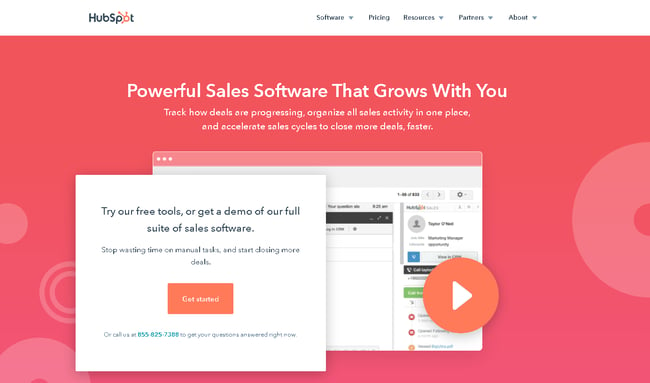The top portion of the image features a white bar with the HubSpot logo prominently displayed. To the right of the logo, the navigation menu items include "Software," "Pricing," "Resources," "Partners," and "About." Beneath this bar is a pink background adorned with light pink circular designs. Dominating the center of the pink background is a bold headline that reads, "Powerful Sales Software that grows with you." Subheadings describe key features: "Track how deals are progressing," "Organize all sales activity in one place," and "Accelerate sales cycles to close more deals faster."

An orange play button is situated below this text, superimposed on a window. A white box beneath the play button offers a call to action: "Try our free tools or get a demo of our full suite of sales software." An orange rectangle labeled "Get Started" is prominently placed in the center, inviting engagement. Below this button is additional text, which is unfortunately too small and blurry to read.